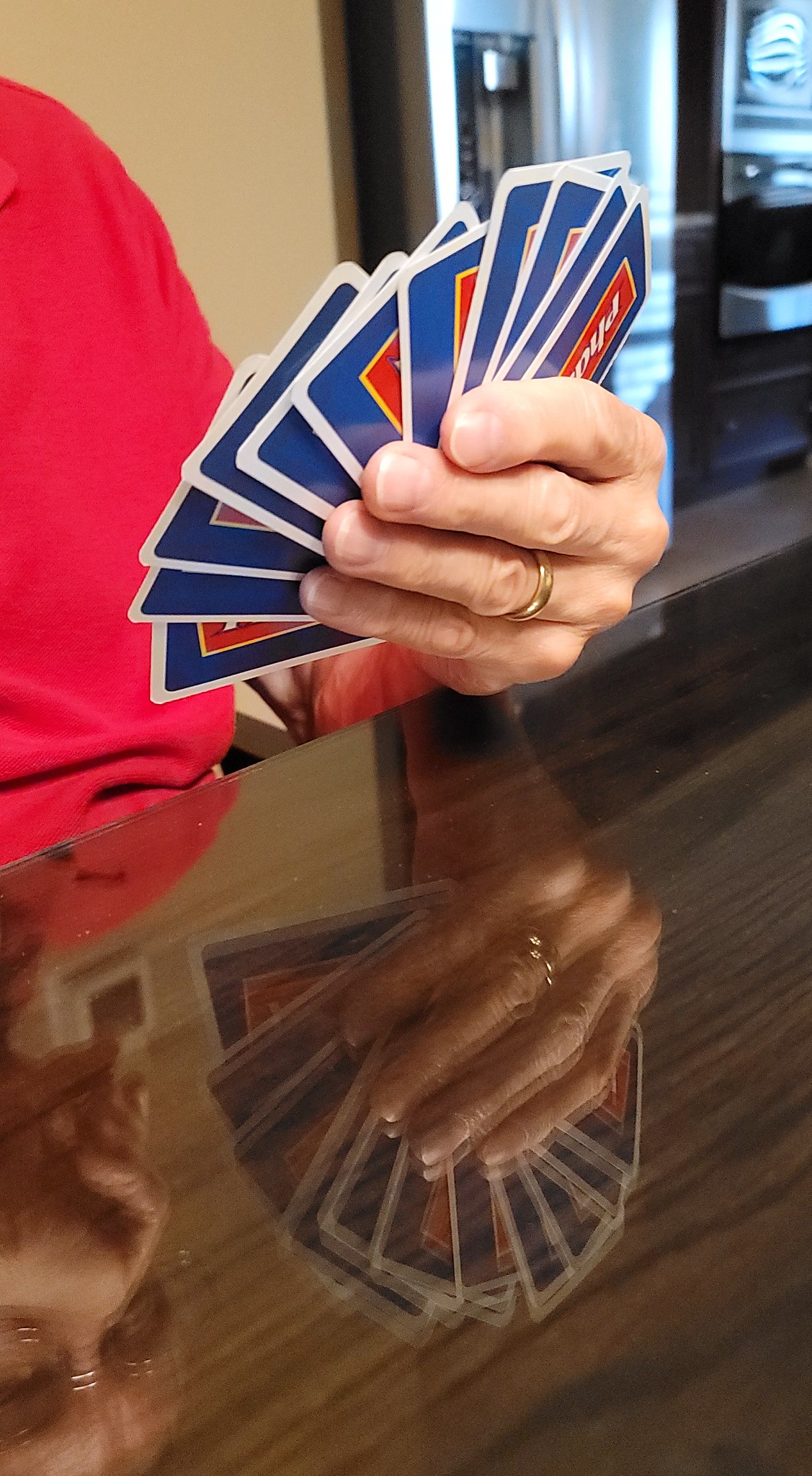In this image, a person is engaged in a game of cards. The individual is positioned on the left side of the picture, slightly below center, with their arms and cards angled upward to the right. They are wearing a red shirt, which drapes down behind their hands and then extends out around the cards, revealing their four fingers, fingernails, and knuckles. A gold band is visible on their ring finger. Part of their elbow rests on a shiny brown table, along with the visible arm of a chair underneath it.

The playing cards are fanned out from the left, with the top card pointing to the left and ascending to the right. The cards have a blue background with a white border and a red rectangle in the center. In the background, a brown wall occupies about a third of the image, ending in dark black trim. There's an opening to another well-lit room, though no details of that room are discernible. To the right of this opening, a brown dresser is faintly visible in the distance.

The table in front of the person is so shiny that their face is reflected upside down in the bottom left corner of the image, revealing that they are wearing glasses. Additionally, just above and to the right of this reflection, you can see a mirrored image of their hand and the spread-out cards.